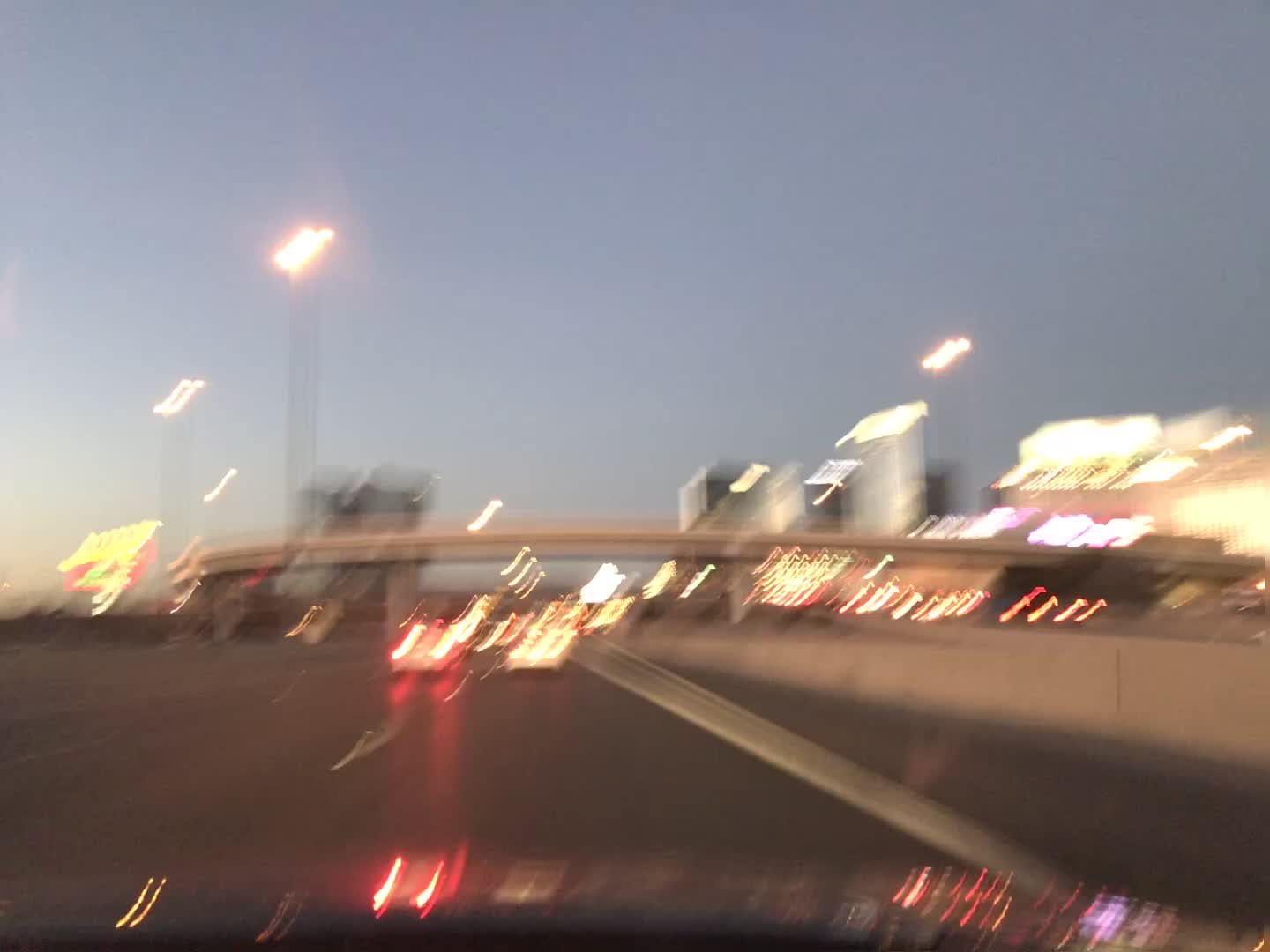The image is a blurry, motion-heavy scene taken from inside a car, with the hood of the car visible in the foreground. The shot is taken so close to the windshield that specific details are hard to make out. The scene is filled with various lights, suggesting the car is driving on the left side of a freeway. In the blurry distance, the taillights of two cars stretch into light trails, enhancing the motion blur effect. The sky is dusky, indicating the sun is setting, casting a dim, transitioning light across the sky. A bridge spans the highway in the background, and a tall metal structure with lights, possibly from a sports field, adds to the illuminated chaos. On the right side of the image, the city's skyline with numerous buildings and glowing lights forms a backdrop, though specific architectural details are indiscernible. A cement divider to the right further grounds the scene within the urban landscape.